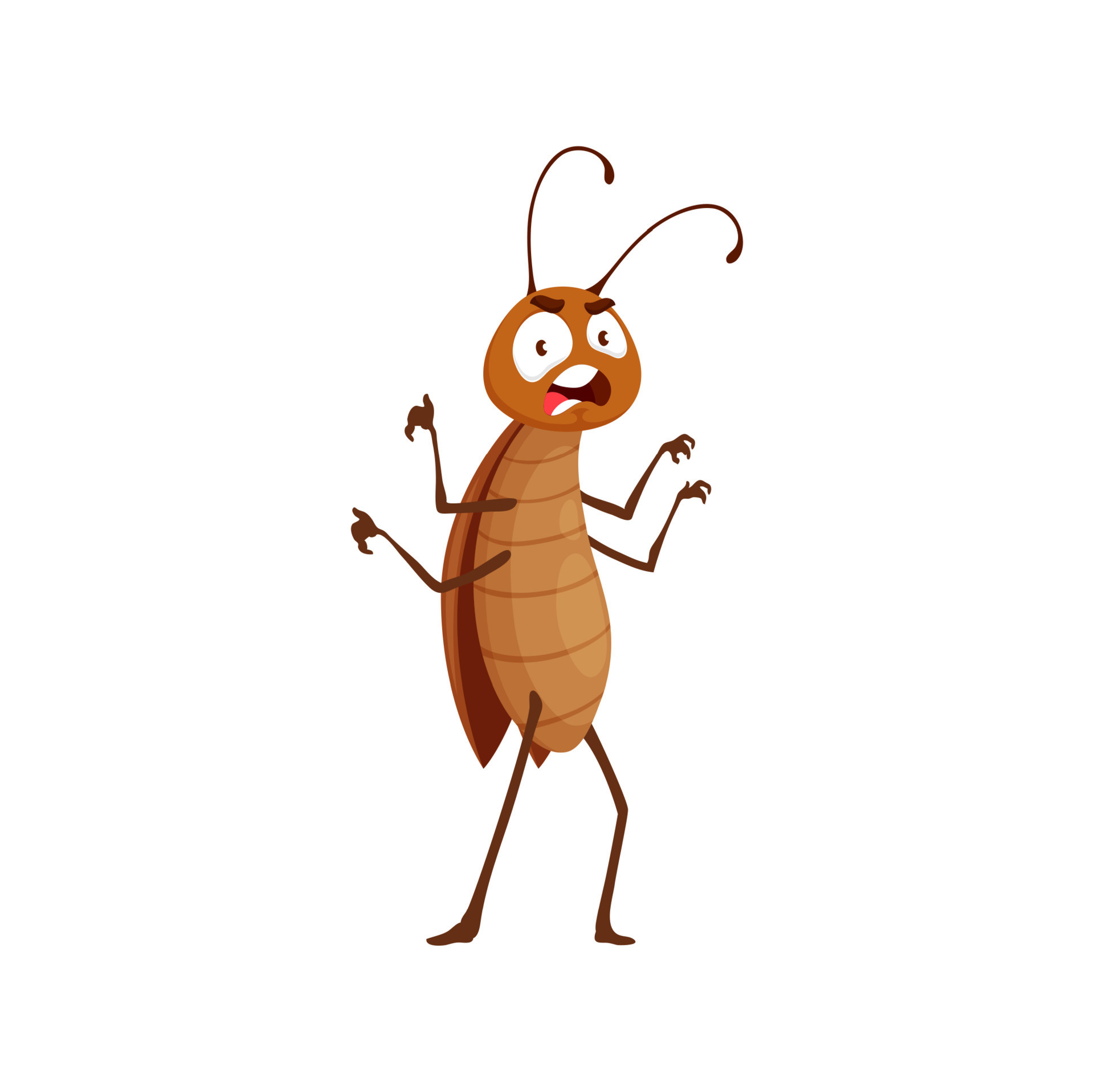The image is a cartoon drawing of an insect, likely a fire ant or a cockroach, with an expressive and exaggerated appearance. Standing upright on two skinny, brown legs, it features a peanut-shaped body adorned with darker brown horizontal stripes. The insect has an amusing yet intense facial expression, combining elements of anger and fright. Its large, white eyes are accented by dark brown eyebrows raised upward, and its wide-open mouth reveals a red tongue and white teeth. The creature possesses four arms, all bent at the elbow and stretched outward as if preparing to defend itself. Two brown antennas protrude from its head, enhancing its animated look. Behind its tan-brown body appears to be a small shell-like structure, and the entire scene is set against a white background.